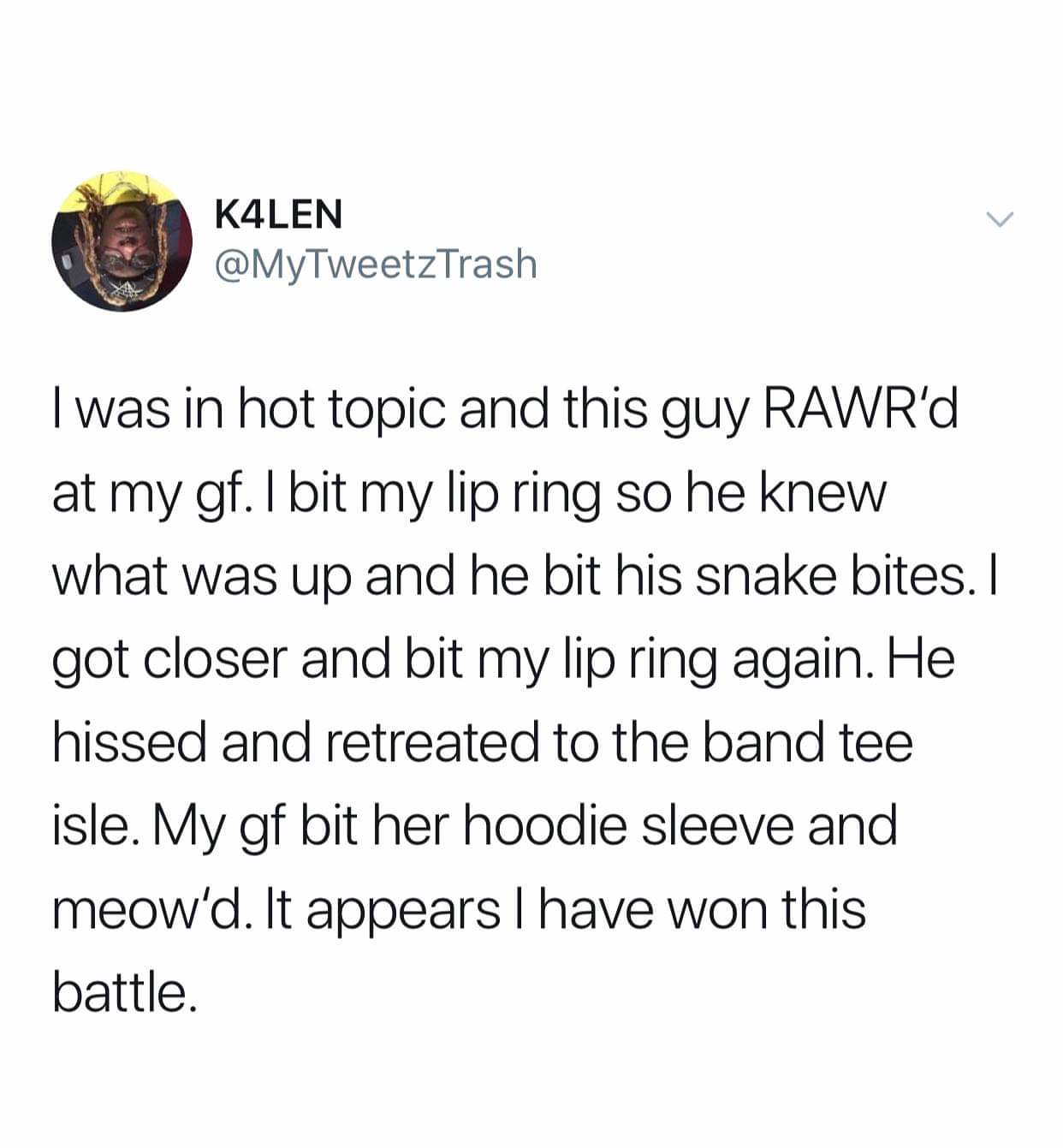This image shows a tweet from a social media post by a user with the handle '@mytweetstrash' and the name 'K4LEN'. The user's profile picture, which is displayed at the top, appears upside down and shows a person with shoulder-length dreadlocks, glasses, and a yellow shirt. The person is wearing a headband that ties at the front. The tweet is in black text against a white background and reads: 

"I was in Hot Topic and this guy r-a-w-r'd at my GF. I bit my lip ring so he knew what was up, and he bit his snake bites. I got closer and bit my lip ring again. He hissed and retreated to the band tee aisle. My GF bit her hoodie sleeve and meowed. It appears I have won this battle."